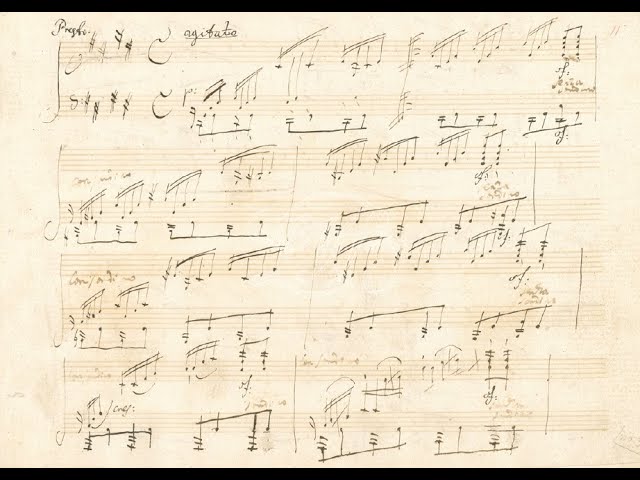The image is an older-looking black-and-white sheet of music. It has a thin black bar at the top and bottom, framing the page. The sheet features horizontal music bars with numerous musical notes, including quarter notes, sixteenth notes, and eighth notes. There are a total of eight horizontal lines, each detailed with vertical and horizontal lines interspersed with small circles representing the musical notes. At the top-left corner of the sheet, there is a cursive text signature that is difficult to decipher, and there are words that look like "adjubate" and "P" or "PRO." The sheet also has a few side notes and annotations about the music itself. The paper appears to have a pinkish background and some handwritten notes, possibly added by someone who was transcribing or annotating the melody. The entire sheet is drawn with what appears to be black pencil, adding to its vintage feel.